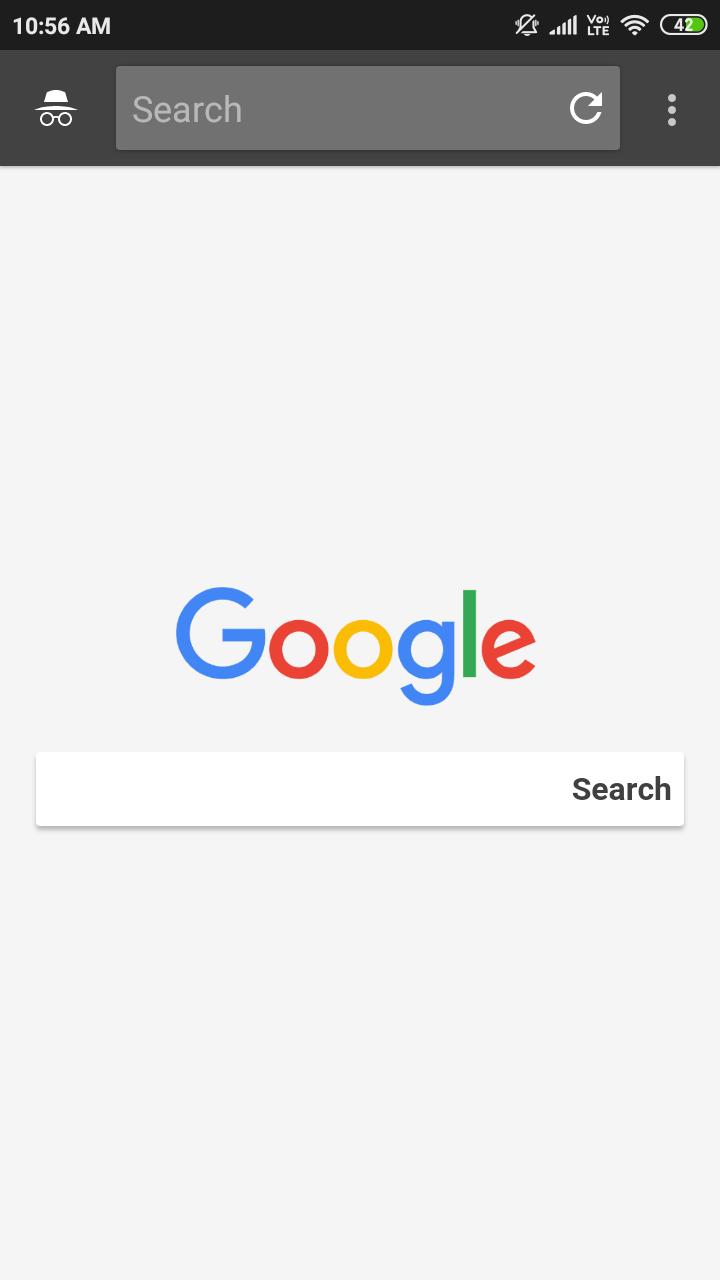A screenshot depicts the Google homepage set against a gray background. The Google logo prominently features the following colors: blue for both G's, red for the first O, yellow for the second O, green for the L, and red for the E. Below the logo, a white search bar displays the word "Search" in black text. In the top-right corner, the time reads 10:56 a.m., and a partially visible battery icon indicates a charge of approximately 42%. The browser is in incognito mode, signified by an icon of a hat and glasses. Additionally, there is a refresh symbol to the right of the search bar, followed by an icon consisting of three vertical dots, which typically denotes a menu or settings options.